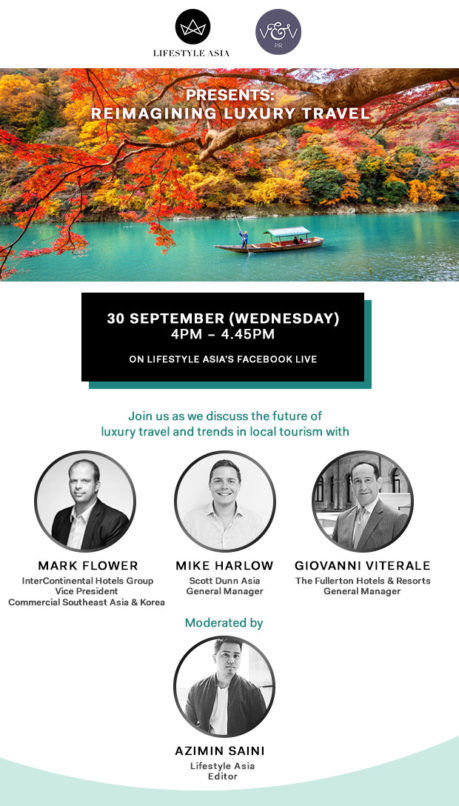The image appears to be a well-designed digital flyer, likely intended for embedding on a website. The design features a clean, primarily white background with very light blue accents and a mixture of black and blue text to complement the accent color. 

At the top of the flyer, there is a picturesque banner showing a serene fall river scene reminiscent of Northeast Vermont, USA, although the setting is Asian as indicated by the website title. In the image, a small boat with an awning is being rowed by an individual standing at the front. The scene is tranquil and inviting.

Above this banner, the text reads "Lifestyle Asia" in a web-interactable button style, though they are static logos. Superimposed on the river scene in white text are the words "presents re-imagining luxury travel."

Beneath the scenic banner, a black square banner overlay with darker blue shading contains the event details. It announces the date "30th September, Wednesday," and the time "4 PM to 4.45 PM" as being hosted on "Lifestyle Asia's Facebook Live." The accompanying blue text invites viewers to "join us as we discuss the future of luxury travel and trends in local tourism with" followed by the names and images of the speakers: Mark Flower, Mike Harlow, Giovanni Viterale, and Azmin Saini. These middle-aged men are pictured in business attire, mostly without ties, except for one gentleman on the right who wears a tie.

Overall, the flyer is an elegant and informative promotional tool, perfectly suited for an audience interested in luxury travel and local tourism trends.